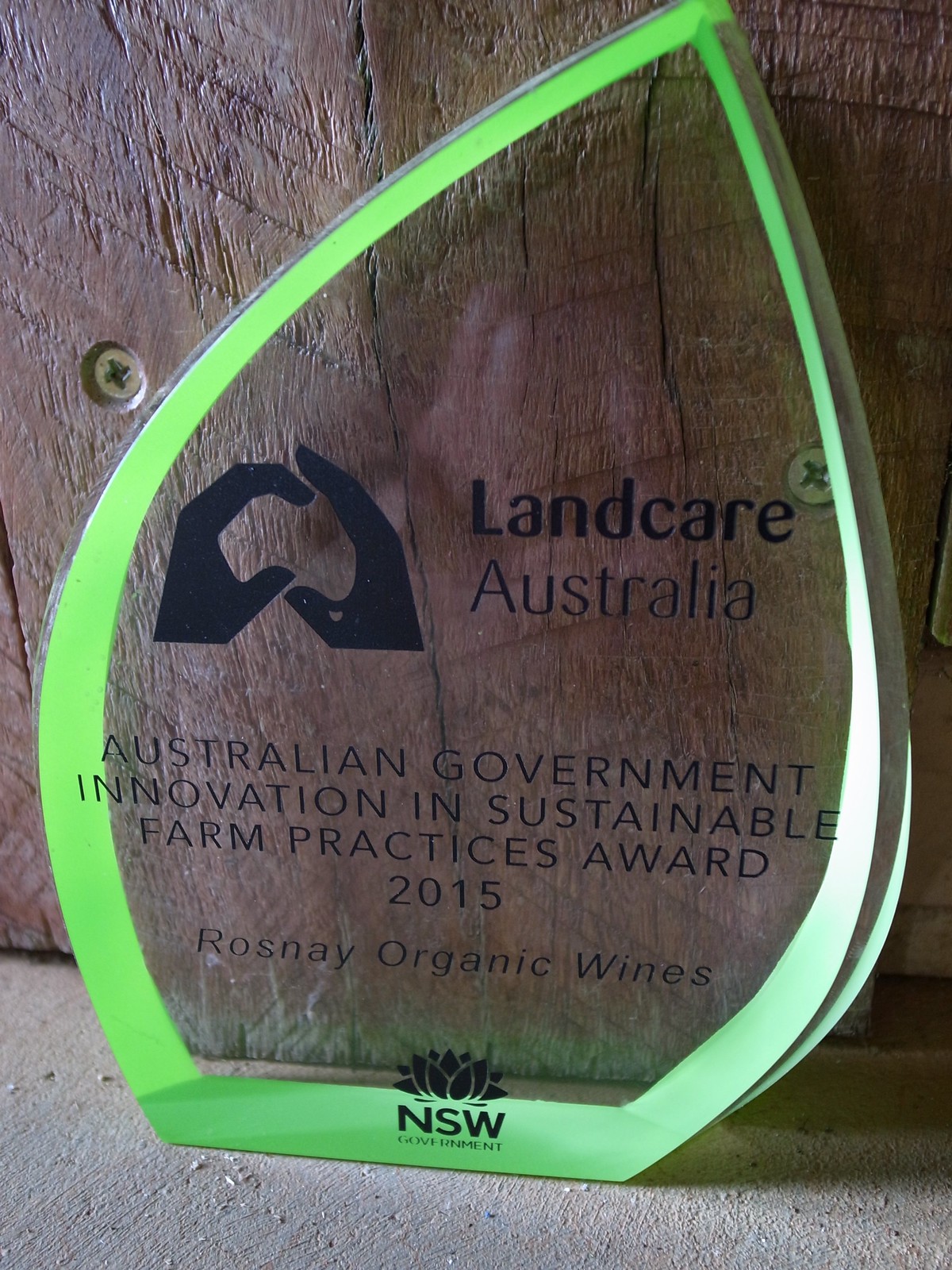The image depicts a transparent glass or acrylic award, shaped like a teardrop or water droplet, with a green outer edge. The setting appears to be outdoors, as the award is leaning against a wooden wall, and the ground beneath it is rough, white concrete scattered with debris. On the award, the left center features an emblem of two cupped hands forming a silhouette resembling the shape of Australia, aligned with Landcare Australia's branding. The right side bears the text "Landcare Australia." Below this, the award is inscribed with "Australian Government Innovation in Sustainable Farm Practices Award 2015," recognizing Rosne Organic Wines. At the very bottom is a lotus flower emblem with the text "NSW Government" beneath it, likely indicating the award's New South Wales origin. The wooden wall behind the award is secured with visible screws, adding to the rustic, outdoor setting.